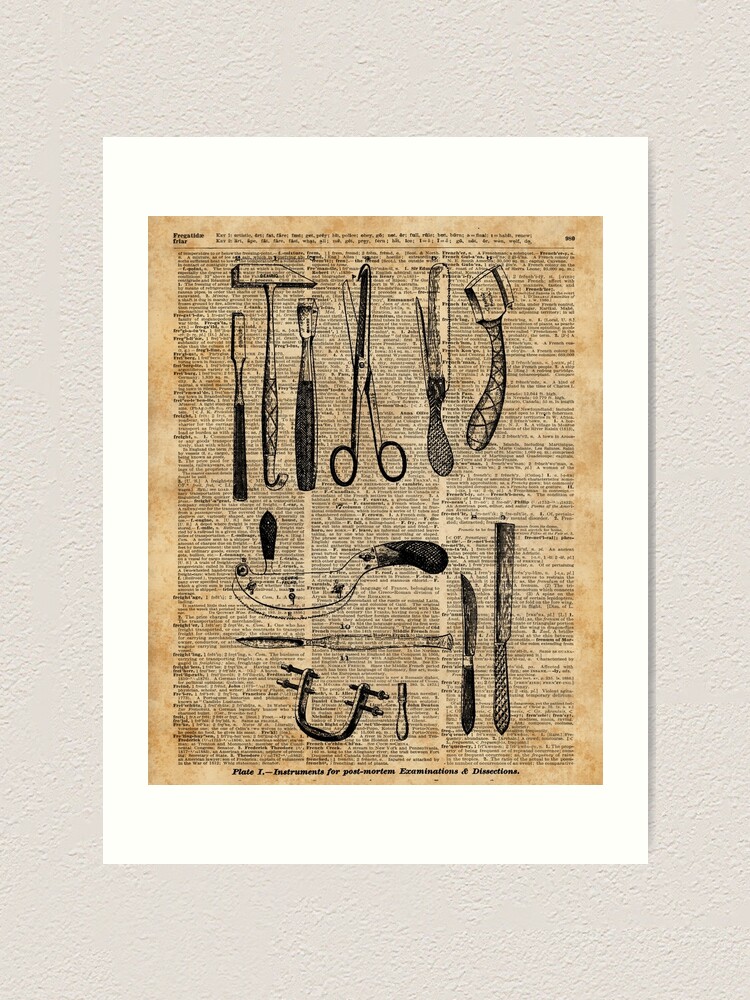This photograph captures a striking vertical print of an old newspaper, which is framed in white and mounted on a textured, off-white wall. The newspaper, a faded light brown in color, serves as the backdrop for a black and white illustration of various tools, most likely associated with post-mortem examinations and dissections, as indicated by the barely legible text on the lower part of the newspaper that reads "Plate one, instruments for post-mortem examinations and dissections."

The illustrated tools are organized into two rows. The top row presents tools in a vertical layout, arranged from left to right: a small wedge, a reflex hammer, another wedge, a pair of scissors, followed by an object resembling a ruler with a curved handle, then a rod, and finally an instrument with a curved handle ending in a razor blade. The bottom row features three horizontally aligned tools: a curved handle tool with a cylindrical protrusion, a pick with a sharp edge, and a U-shaped tool with bolts on either side. To the right of these, there is a vertically positioned knife and a file or razor blade. The intricate details and antique feel of the illustrated instruments contrast beautifully with the small, unreadable columns of text, giving the impression that these tools are part of a historical medical examination set.